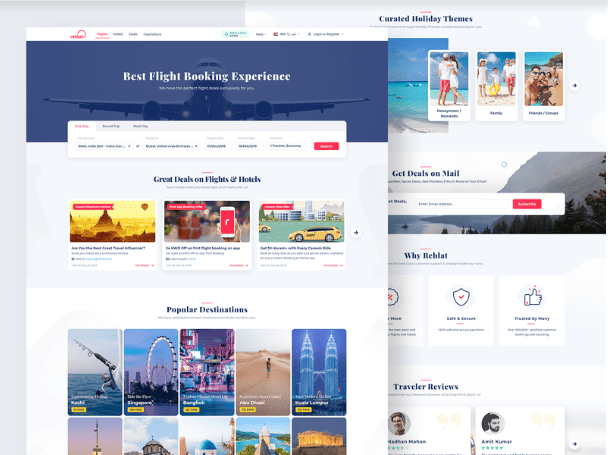In the image, two overlapping webpages are prominently displayed, indicating they pertain to booking experiences, most likely related to travel or vacations. The webpage on the left, partially overlaying the one on the right, proudly features the title "Best Flight Booking Experience." It highlights a striking image of an airplane taking off towards the viewer, symbolizing the start of a journey. Scattered across this site are numerous images showcasing various global attractions, suggesting a focus on diverse travel destinations.

The webpage on the right, which is slightly obscured, centers around a prominent search bar, inviting users to begin their search for travel services. Several clickable links are also visible, hinting at different options or categories available for the user. Both webpages share a clean, white-light themed background, enhancing readability and user engagement. This detailed setup portrays a sophisticated platform designed to facilitate seamless flight bookings and vacation planning.